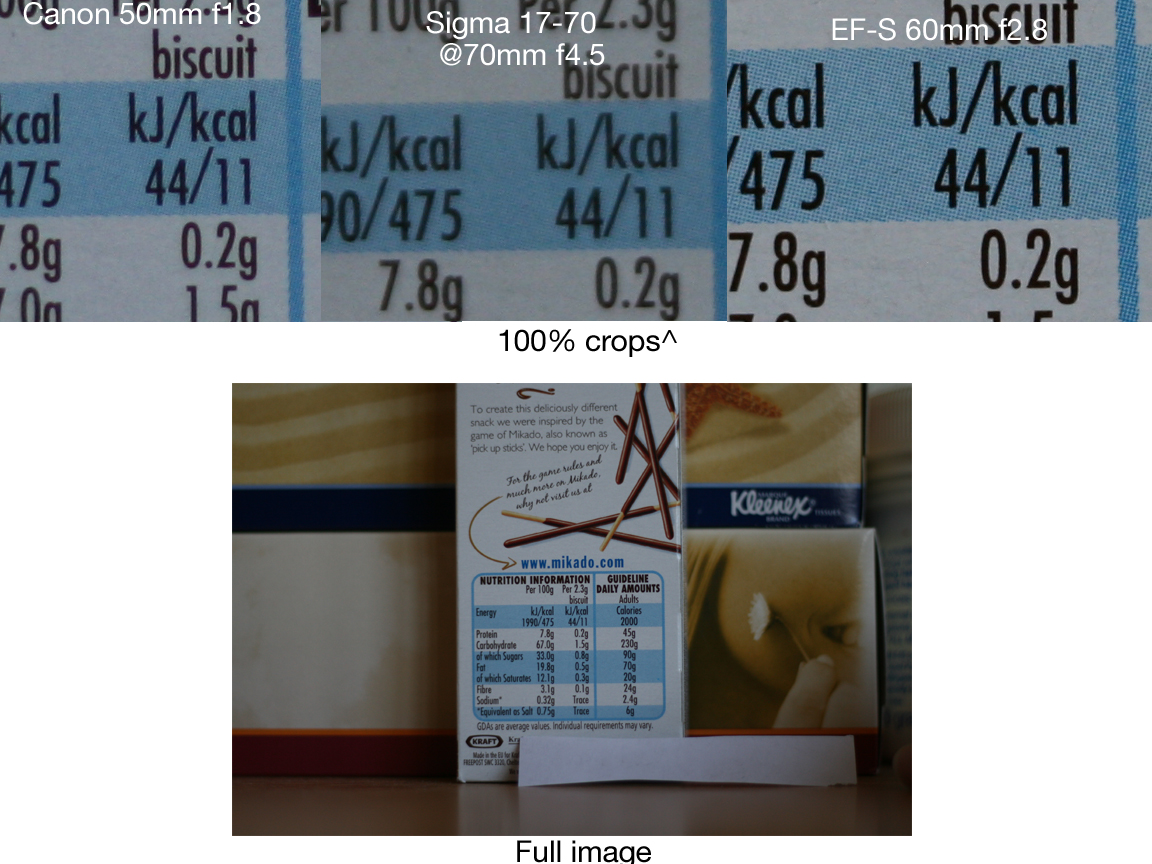This detailed infographic comprises multiple photographs meticulously arranged to present the nutrition facts of a food product. The top row features three distinct images, each representing a different flavor variant, labeled "Canon," "Sigma," and "EFS." Each of these images highlights key nutritional information, particularly focusing on the calorie count, denoted as "kcal." The bottom photograph offers a comprehensive view of the product's label, including a full list of nutrition facts, an image of the food item, and a website URL, www.mikado.com, for further reference. This layout not only provides a clear comparison of the nutritional profiles for each flavor but also ensures that viewers have access to all relevant dietary information at a glance.